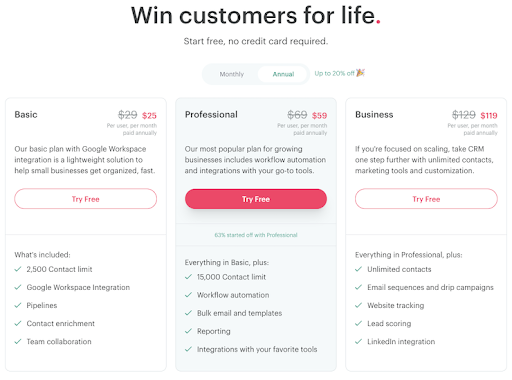The image features a promotional pricing table for a customer management platform, prominently displaying an inviting message at the top center: "Win customers for life" in bold black text. Just beneath this, a smaller, reassuring note reads: "Start free, no credit card required." Below, two selection bubbles labeled "Monthly" and "Annual" are presented, with "Annual" currently selected and accompanied by a note stating "up to 20% off" alongside a celebratory party hat icon.

The pricing table comprises three plans, each described in detail:

1. **Basic Plan:**
   - Price: $25/month (discounted from $29/month)
   - Description: "Our basic plan with Google Workspace integration is a lightweight solution to help small businesses get organized fast."
   - Button: "Try free"
   - Features:
     - 2500 contact limit
     - Google Workspace integration
     - Pipelines
     - Contact enrichment
     - Team collaboration

2. **Professional Plan:**
   - Price: $59/month (discounted from $69/month)

3. **Business Plan:**
   - Price: $119/month (discounted from $129/month)

Each plan's features and discounts are clearly delineated, catering to varying levels of business needs and highlighting the integration with Google Workspace to facilitate organization and collaboration.